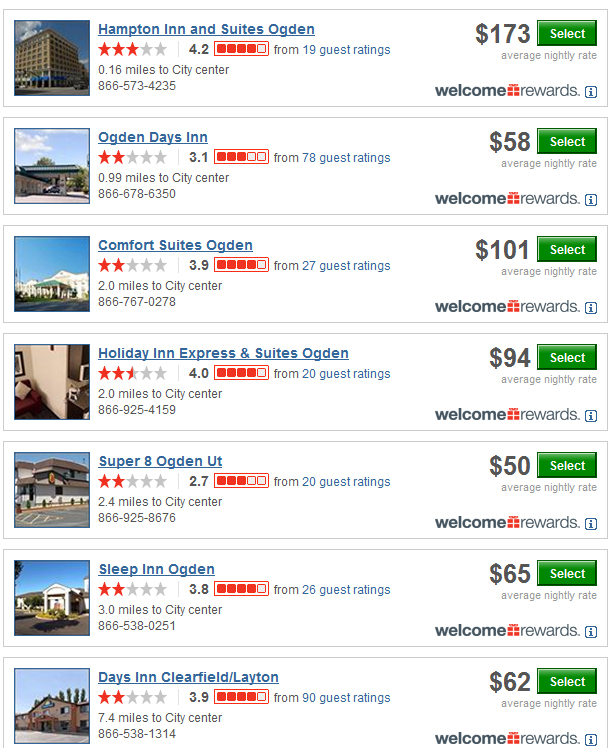Here is the cleaned-up and detailed caption:

---

This image is a snippet from a hotel booking website named "Welcome Rewards." The website aggregates various hotel listings, providing comprehensive details for each option. The layout features seven horizontal boxes, each showcasing a different hotel available for booking. The highlighted details include guest ratings, proximity to the City Center (the searched location), phone numbers, an image of the hotel, the hotel's name, the average nightly rate, and a select button for booking. The website's logo, "Welcome Rewards," is distinctively separated by a present-shaped icon.

The listed hotels are as follows:
1. **Hampton Inn and Suites Ogden**: $173 per night, 0.16 miles from City Center.
2. **Ogden Days Inn**: $58 per night.
3. **Comfort Suites Ogden**: $101 per night.
4. **Holiday Inn Express and Suites Ogden**: $94 per night.
5. **Super 8 Ogden UT**: $50 per night.
6. **Sleep Inn Ogden**: $65 per night.
7. **Days Inn Clearfield/Leighton**: $62 per night, 7.4 miles from City Center.

The hotels are organized based on their distance from the City Center, with the closest being Hampton Inn and Suites at 0.16 miles and the farthest being Days Inn Clearfield/Leighton at 7.4 miles away.